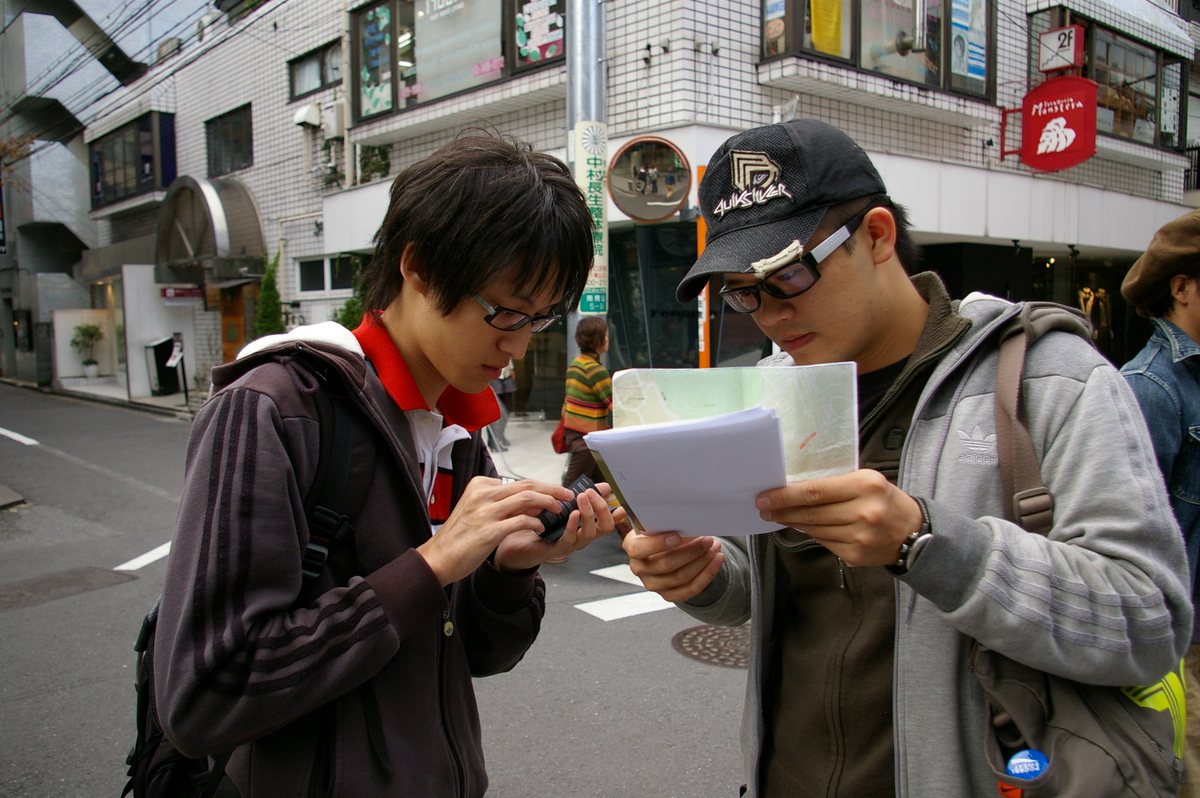In the foreground of the image are two young Asian men standing on a narrow street corner, likely tourists given their focused attention on navigation tools. The man on the left, wearing a brown jacket over a red shirt and sporting a backpack, appears to be using a smartphone, possibly inputting map coordinates. He has medium-length black hair and wears black plastic-framed glasses. The man on the right, dressed in a gray sweatshirt with white Adidas stripes, a black baseball cap featuring a logo, and a tan backpack slung over one shoulder, is holding a sheet of paper that looks like a map along with a notebook. Both men wear glasses, with the second man's glasses featuring white earpieces and black frames. They are surrounded by white-tiled buildings which extend halfway down the block on the left and continue to the right as far as the photo allows. An illegible sign is visible between their heads, and Asian characters on nearby signs suggest the setting is in a non-U.S. Asian town. The street is marked for traffic, but no sky is visible in the frame.